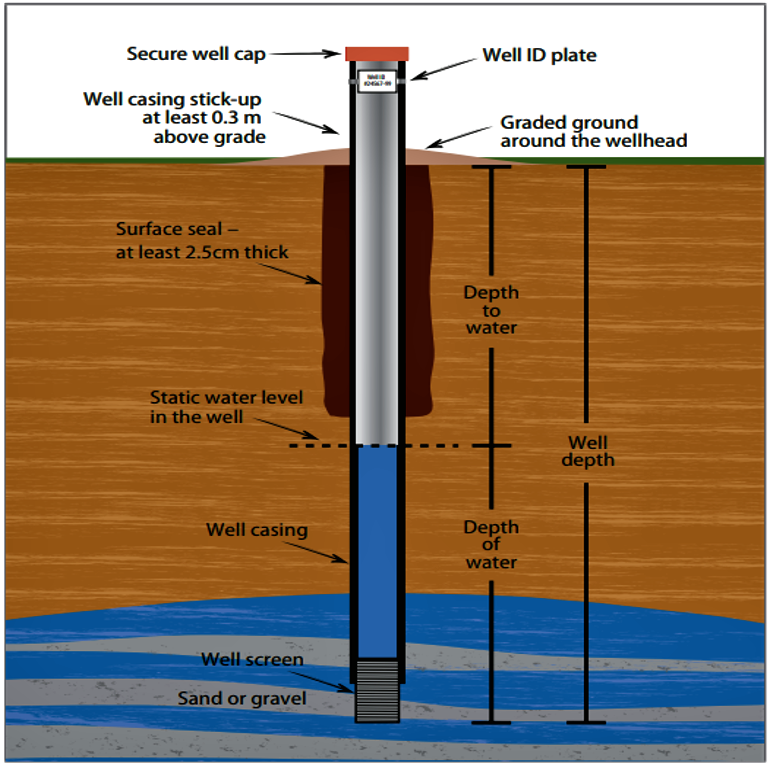This detailed infographic illustrates the structure and components of a well system extending from the earth's surface into the water below. The diagram is segmented into three color-coded zones: a white area at the top representing the surface, a brown area in the middle symbolizing soil, and a blue-gray area at the bottom depicting water.

At the very top of the well structure, there is a secure, red well cap. Directly beneath it, a white well ID plate with prominent lettering is attached. The well casing extends from at least 0.3 meters above the surface level (graded ground) down through the soil, penetrating into the water layer below.

The graded ground around the well head ensures stability, while a surface seal, at least 2.5 centimeters thick, provides additional protection. As one looks further into the well, various annotations mark critical depths, including the depth to water and the static water level.

The well casing, depicted in blue, traverses from the silver-colored upper portion down into the water. At the bottom end of this casing lies the well screen, allowing water to enter while filtering out debris, and surrounding sand or gravel acts as a further filtration medium. The infographic highlights key measurements and labels such as the well depth, depth of water, and the static water level within the well, providing a comprehensive overview of a well's anatomy and functionality.